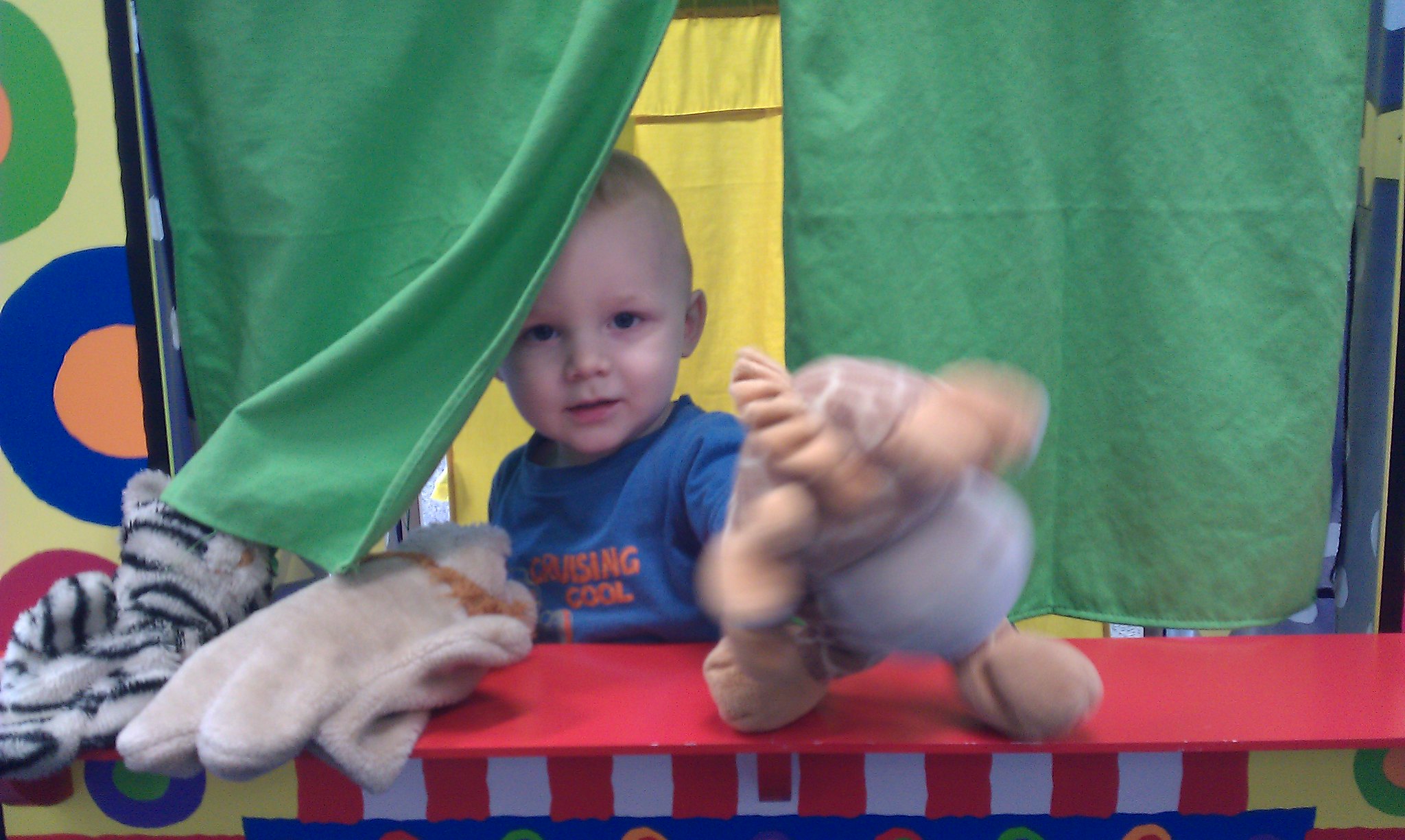The image depicts a young boy, approximately one or two years old, with fair skin and short fair hair, standing behind a vibrant, colorful booth that resembles a puppet show stage. The booth features green curtains, a top with red and white stripes, and a decorative red front shelf. The boy, wearing a blue t-shirt with the words "Cruising Cool" in orange letters, is peering through the curtains while engaging with a hand puppet. He appears to be manipulating a hand puppet that is somewhat blurred, possibly resembling a chicken or dinosaur with white, brown, and splotchy details. To the left side of the booth, several other hand puppets are visible, including a black-and-white striped cat and a light-colored animal, potentially a lion or another ambiguous creature. The background behind the boy is yellow, adding to the overall vibrant and playful setting, which evokes the charm of a children's puppet show or play area. The boy is looking directly at the camera, capturing a candid moment of childhood curiosity and play.